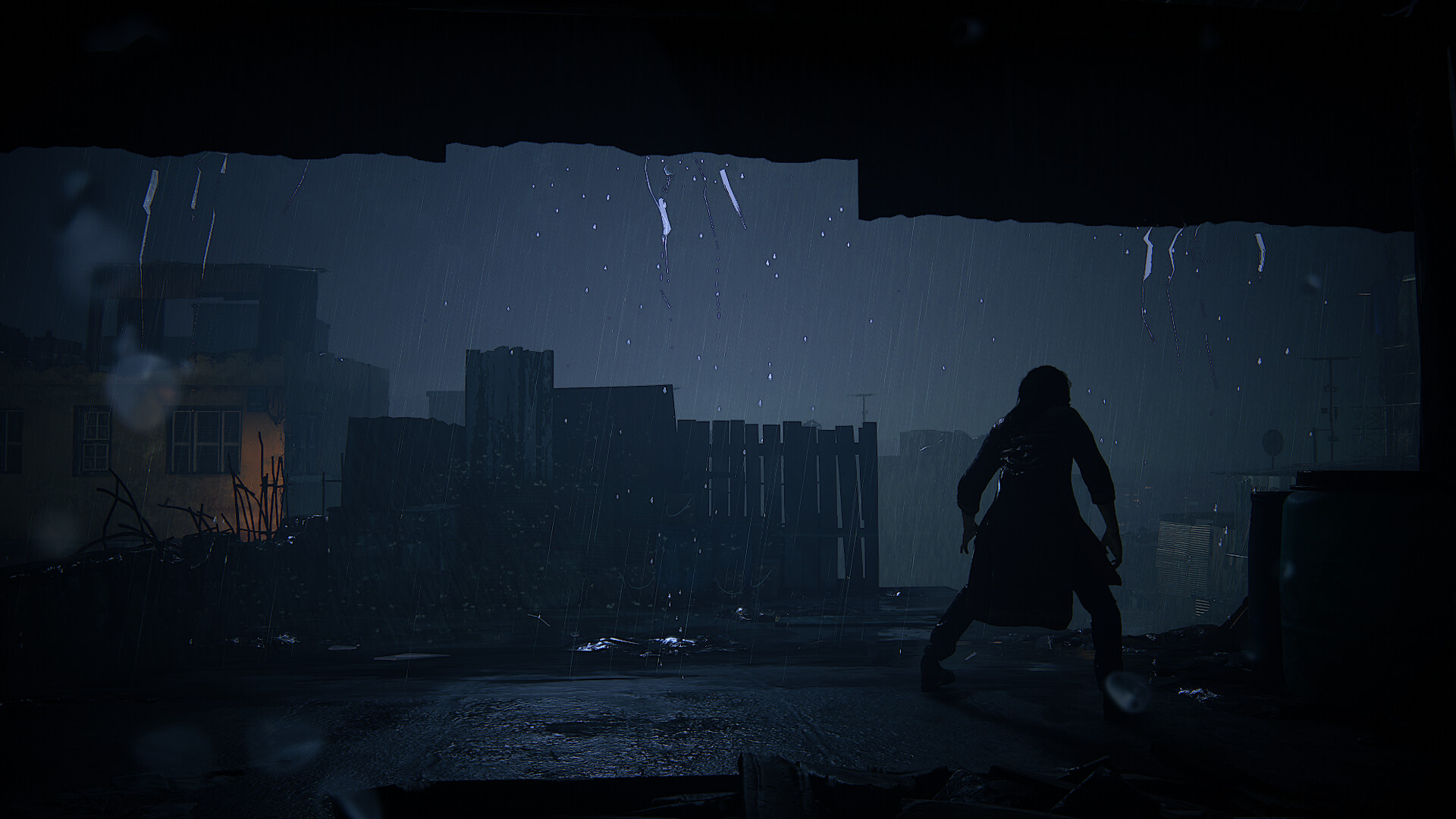This image, potentially a screenshot or concept art for a video game, movie, or comic book, showcases a distinctive visual style blending realism with cel-shaded, cartoon-like elements. The scene is imbued with a dark, moody atmosphere, dominated by a navy-colored sky at the top, suggesting a nighttime or stormy setting. Rain lightly drizzles from above, adding to the dramatic ambiance. White and light blue cel-shaded lines dangle from rafters above, intensifying the stylized aesthetic.

At the center of the image is a character outlined in black, hunched over in a lunge-like position, hinting at stealth or tension. The ground is depicted in dark gray, slick with rain, enhancing the sense of wetness and gloom. In the background, a wooden fence is also rendered in black outlines, contributing to the stark, graphic quality of the art. A slight orange glow emanates from a building off to the left, providing a subtle contrast and focal point in this otherwise dark and brooding composition.